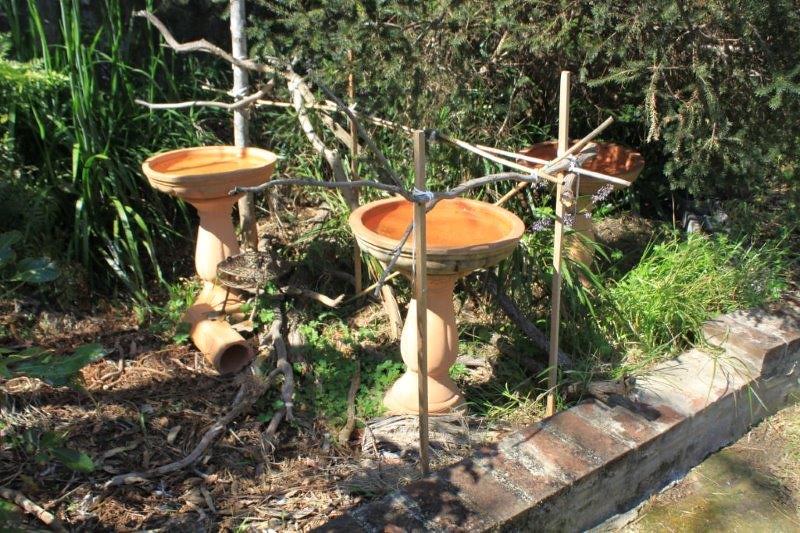This daytime outdoor image depicts an unkempt garden or yard featuring three prominently visible birdbaths, though the third is only partially discernible. The birdbaths are matching structures, made of a light beige material resembling concrete and are shaped like large basins supported on bases reminiscent of pawn chess pieces. Each birdbath is filled with water tinged with an orange hue. Surrounding the birdbaths is a mix of overgrown and dead vegetation, with clusters of weeds, fallen twigs, and brown, dead grass scattered on the ground. Encircling the birdbaths is a roughly constructed fence made from wooden stakes and natural-looking sticks arranged in an oblique X-pattern and horizontal rails. In the lower right-hand corner, there is a section of mortared brick garden edging several inches high, which is old, worn, and faded, forming a slight pathway. The background is rich with trees and shrubbery, enhancing the garden's lush yet untidy ambiance.